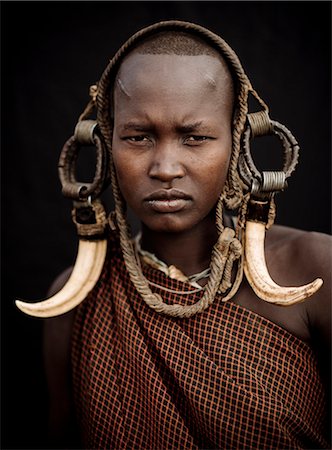This is a striking portrait of a young African woman set against a completely black background, drawing full attention to her intense and serious expression. She gazes directly into the camera, her dark brown eyes underscored by a slight furrow in her brows. Her skin is a rich, dark tone with an even complexion, and her head is adorned with a short, shaved haircut. Notable are the scars on her forehead, one on each side, adding to her distinctive appearance.

She wears a unique headdress that appears to be made of leather or rope, encircling her head and extending below her chin. From this headdress dangle large circular ornaments near her ears, attached to which are curved bones or tusks, suggesting animal origins. These adornments curve downward and outward, creating a striking frame for her face.

Her attire consists of a draped, one-shoulder outfit, predominantly black with orangish-red stripes, elegantly exposing her right shoulder while covering her left shoulder. The fabric could be described as a toga-like material, adding to the traditional and cultural essence of her appearance. The overall visual impact is one of deep cultural significance and solemn beauty.